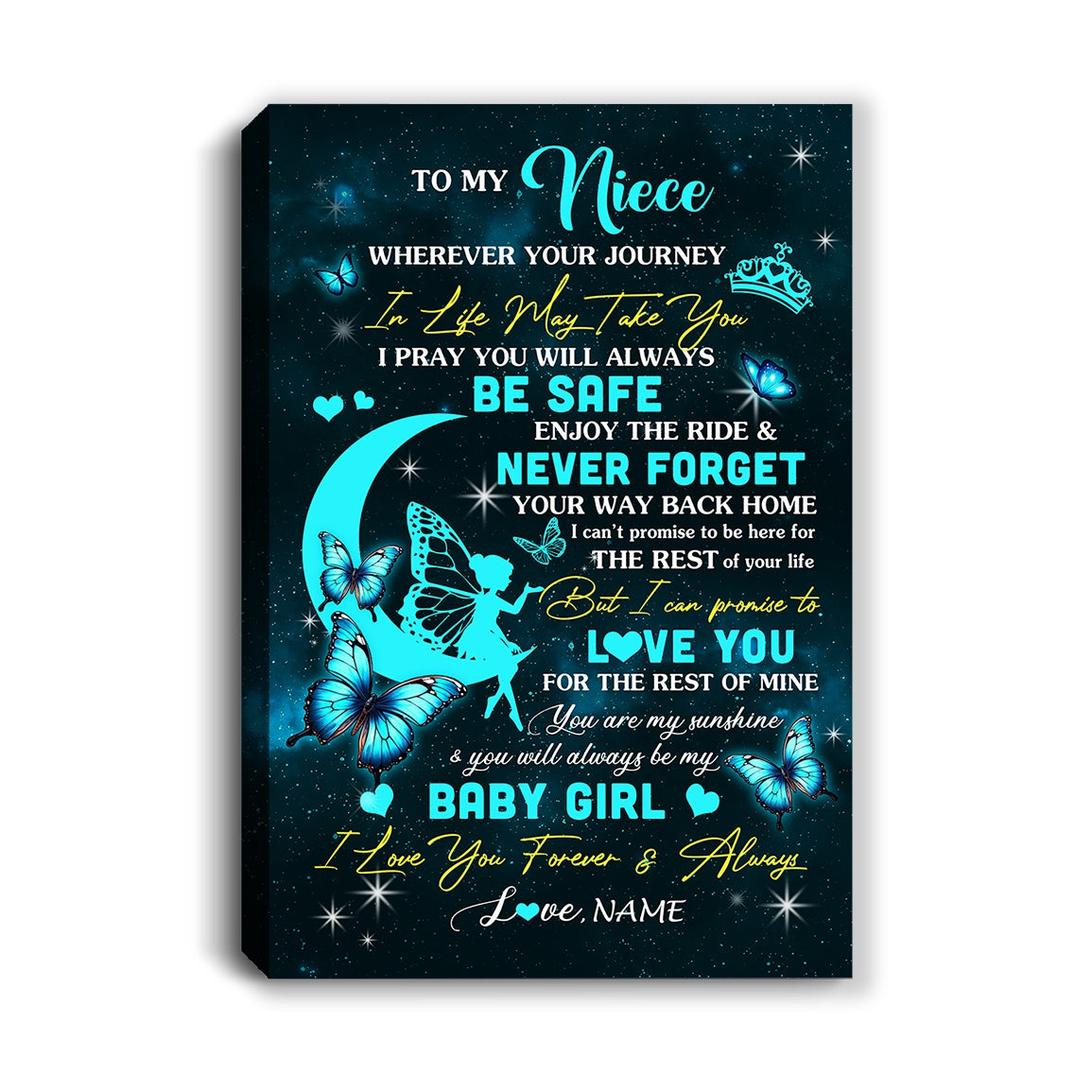The image features a beautifully crafted wall art, likely designed to be a heartfelt gift for a niece. Set against a dark blue to almost black background that evokes the night sky, the center showcases an affectionate message in a mixture of white and teal lettering. The text reads: "To my niece, wherever your journey in life may take you, I pray you will always be safe. Enjoy the ride. Never forget your way back home. I can't promise to be here for the rest of your life, but I can promise to love you for the rest of mine. You are my sunshine and you will always be my baby girl. I love you forever and always. Love, [Name]."

The art is adorned with various fantasy-themed elements. Small to large white stars are scattered throughout the background, enhancing the celestial feel. Teal and light blue butterflies add a whimsical touch, one prominently positioned at the bottom. To the left of the text, a half-moon features a fairy-like woman sitting on its edge, with delicate butterfly wings. A princess crown with a teal accent is placed towards the upper right. A few teal hearts are also interspersed within the design, contributing to its charming and dreamy aesthetic. This personalized piece is perfect for adorning a young girl's room, symbolizing an aunt's enduring love for her niece.